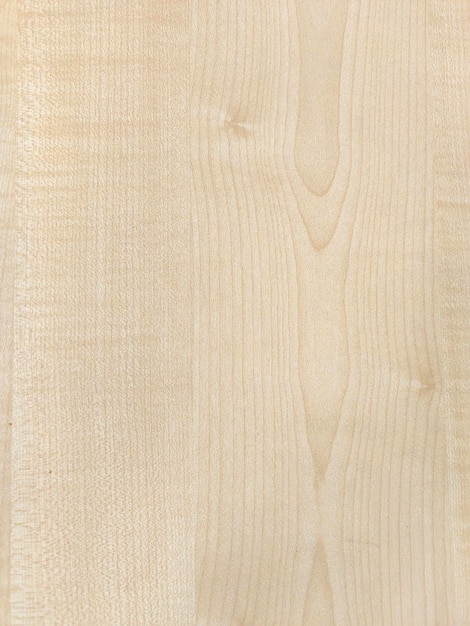This image features a rectangular panel of very light-colored wood, almost a grayish-white, measuring approximately 30 to 40% taller than it is wide. The wood's surface is notably smooth with vertical grains running from top to bottom. The panel's left third showcases tightly packed grains, while the grains spread further apart and grow thicker as you move towards the right side, culminating in the thickest grains about 70% across the width. This thickest section features grains that resemble vertical cells, some of which are darker shaded. The far right edge, constituting about 5% of the width, reverts to thinner grains. The wood also displays a significant knot near the top center, with dark brownish rings emanating from it in a diagonal pattern. This knot, along with the darker edges, provides striking contrast against the predominantly light wood, which is lighter than typical tan or brown shades. There are no other elements or objects around the wood in the image, and the wood appears two-dimensional due to the lack of visible depth.